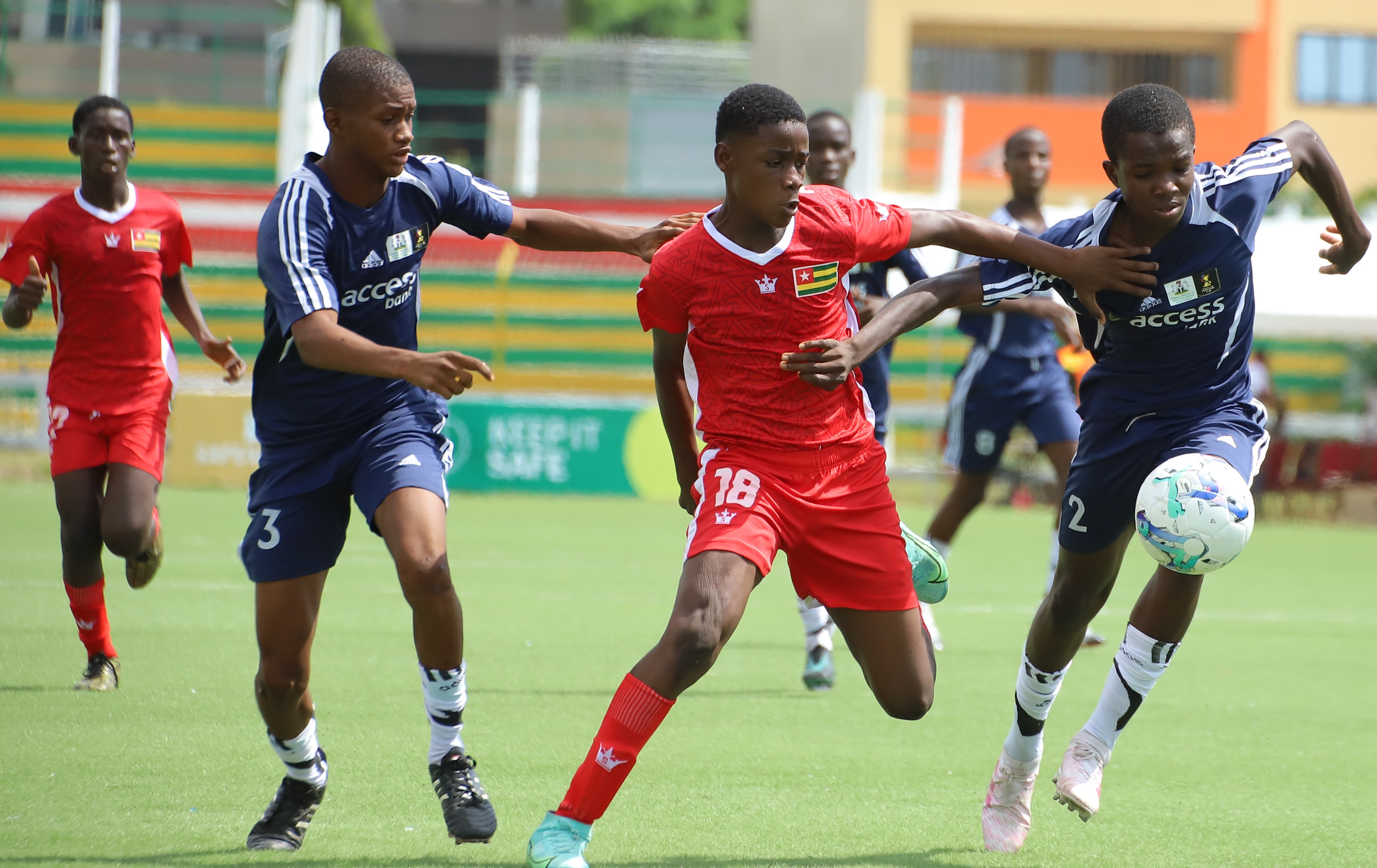This detailed outdoor photograph, taken during the daytime, captures six young African descent men playing soccer in a stadium covered with vivid green grass. The players are split into two teams. The team in red sports short-sleeved jerseys and knee-high socks adorned with white crowns at the bottom of the neck collars. One red team player's jersey features the number 18 on his right leg. The opposing team wears dark blue uniforms with three distinctive white stripes along the sleeves, and the word "ACCESS" printed across their chests. Players in blue also wear knee-high socks and have the Adidas logo on their apparel, with some players displaying the numbers 2 and 3 on their legs. 

In the action shot, a player in blue on the right clutches a teammate's arm as they both chase after a white soccer ball marked with blue and green designs. Their shadows stretch to the left, cast by the sun above. Beyond the pitch, the boundary fence is adorned with banners, and some blurred buildings are visible in the background, adding depth to the scene.